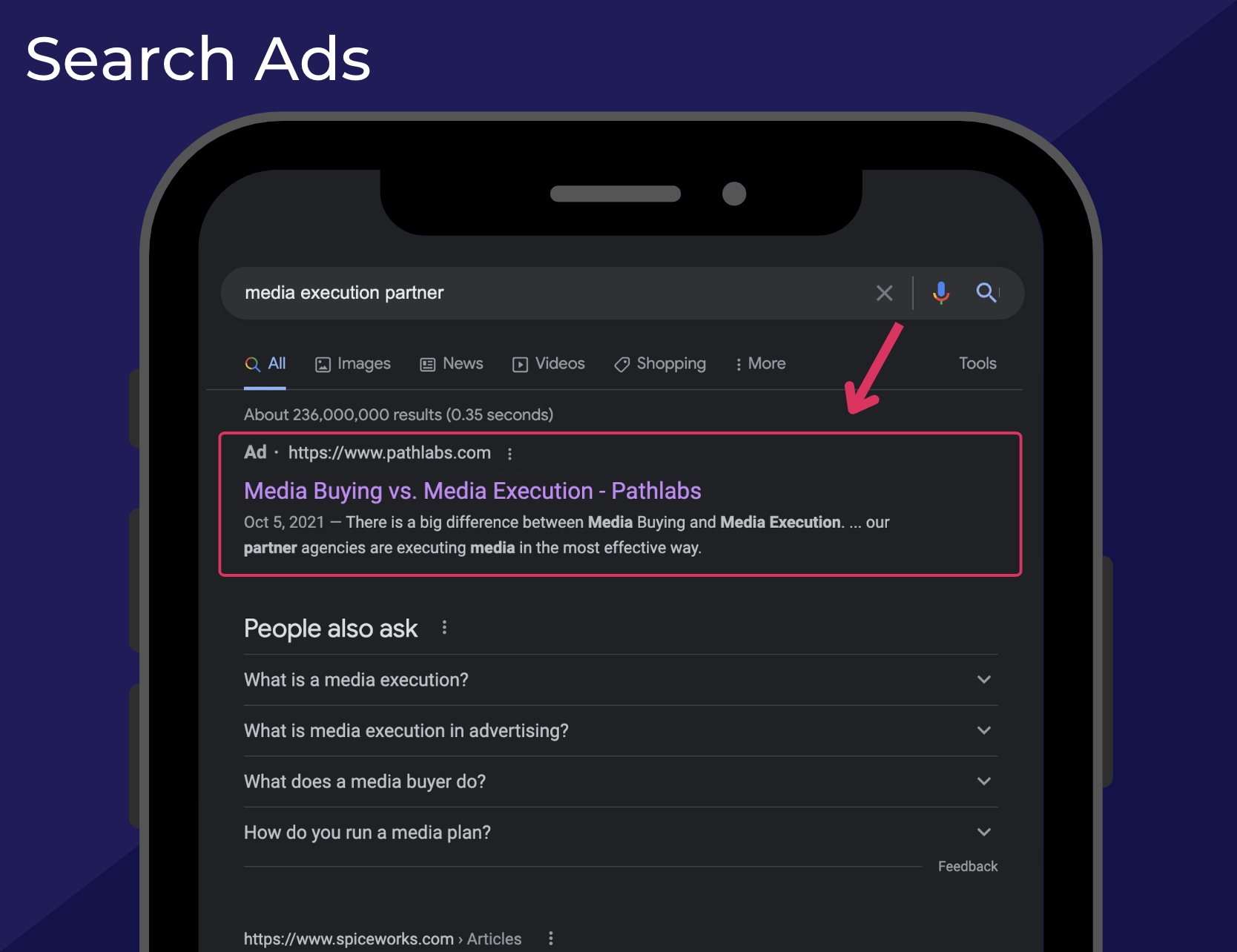A digital screenshot featuring a mobile phone interface with a vibrant blue background. The focal point of the image is a search engine results page with several elements displayed in white. At the top of the screen is a prominent search bar flanked by icons – an 'X', a microphone, and a magnifying glass. Just below the search bar, the interface displays various filter options including "All," "Images," "News," "Videos," "Shopping," and "More," with the "All" option highlighted in blue.

Prominent within the search results is an advertisement titled “Media Buying vs. Media Execution - Path Labs.” The ad's publication date, October 5, 2021, and a brief description that emphasizes the importance of effective media execution by partner agencies are also visible. This content is enclosed within a conspicuous red rectangle, which is accompanied by a red arrow pointing directly to the ad, emphasizing its significance.

Beneath the ad, a section titled "People also ask" includes suggested queries like "What is media?", "What is a media execution?", "What is media execution in advertising?", "What does a media buyer do?", and "How do you run a media plan?". The search page indicates that there are about 236 million results, retrieved in approximately 0.35 seconds.